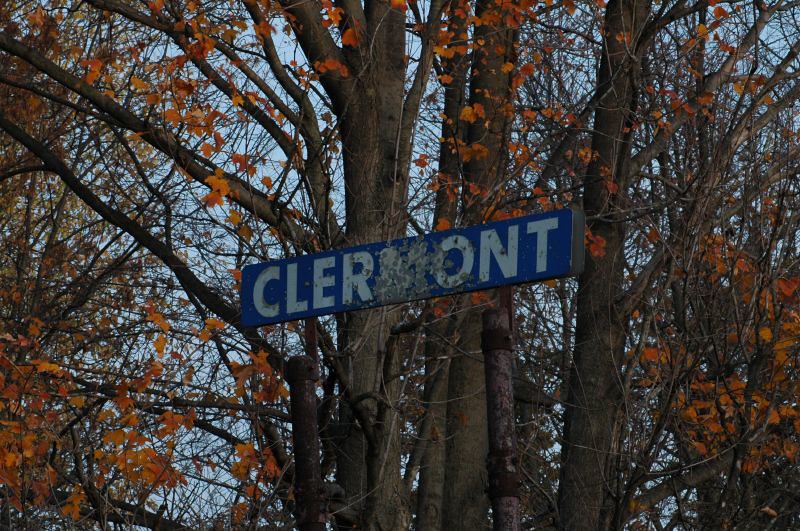In this photograph, a blue sign displaying the word "CLERMONT" in capitalized, white letters is securely mounted on a multi-trunk tree. The tree appears to be quite distinctive, with several trunks branching out and extending upwards. Surrounding the tree are numerous orange leaves, suggesting that the image was taken during the fall season. The sky in the background is a vivid, clear blue, adding a crisp contrast to the autumnal colors. The scene is serene and picturesque, capturing the essence of a peaceful fall day.